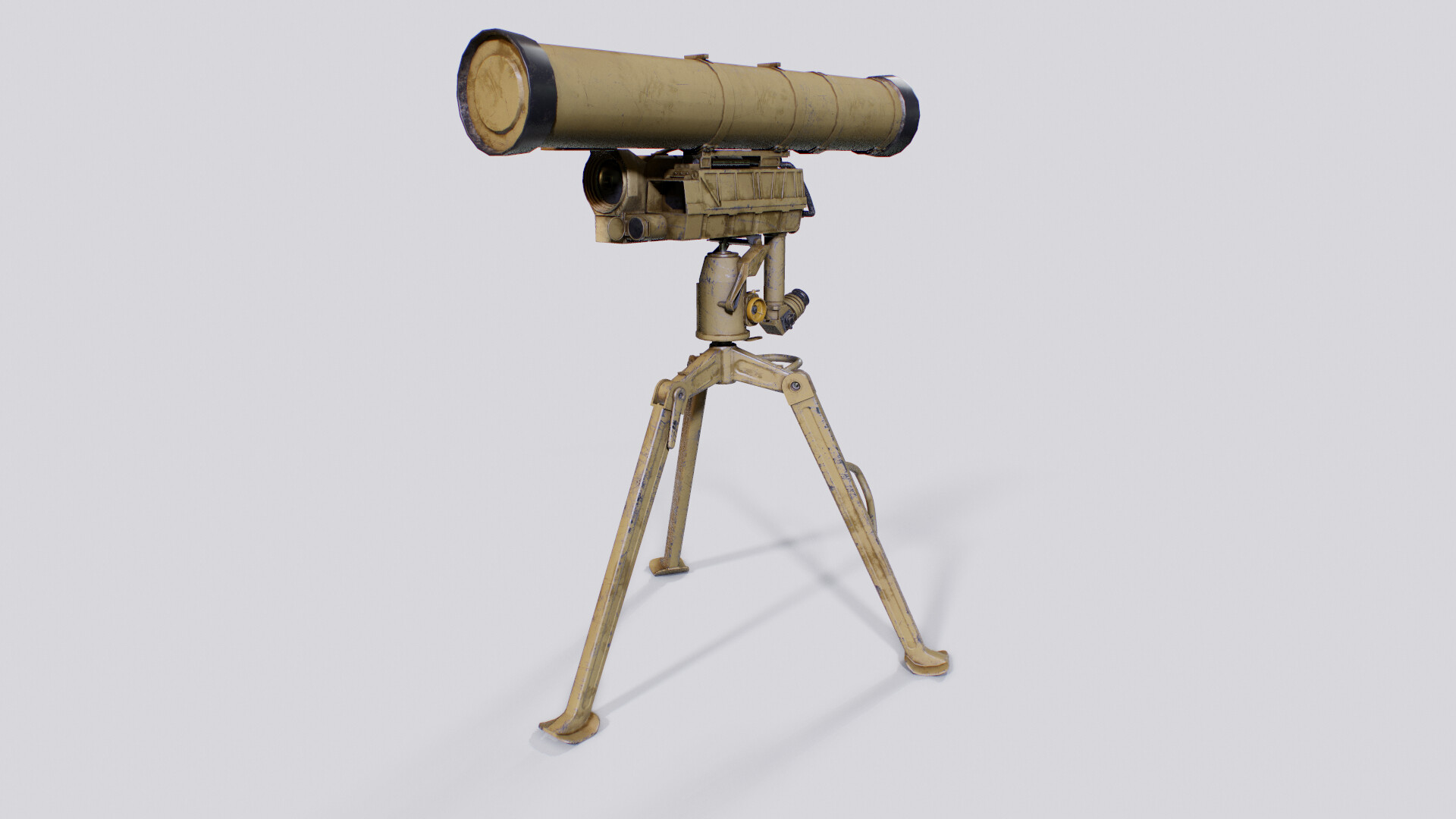The image is a detailed color photograph taken indoors, displaying a vintage piece of equipment on a tripod. The central object appears to be an old, military-style telescope, although there is some ambiguity regarding its precise function; it could potentially be a measuring instrument or, less convincingly, a type of firearm. Both the telescope and the tripod are painted in a weathered cream color, resembling a light tan or military olive drab, with black bands capping the ends of the telescope's long cylindrical body. The telescope is oriented facing the left side of the image with the viewer portion on the right. Beneath the main cylinder, there is a smaller section with a circular lens on the left-hand side and a more box-like structure on the right, possibly for calibration. The entire setup, including the tripod, stands firmly on three metal legs, with an adjustment lever under the rectangular unit. The background is a plain, light gray, situating the equipment clearly in the center of the photograph, which is in landscape orientation and measures about six inches wide by three inches high. The style is photographic representational realism.